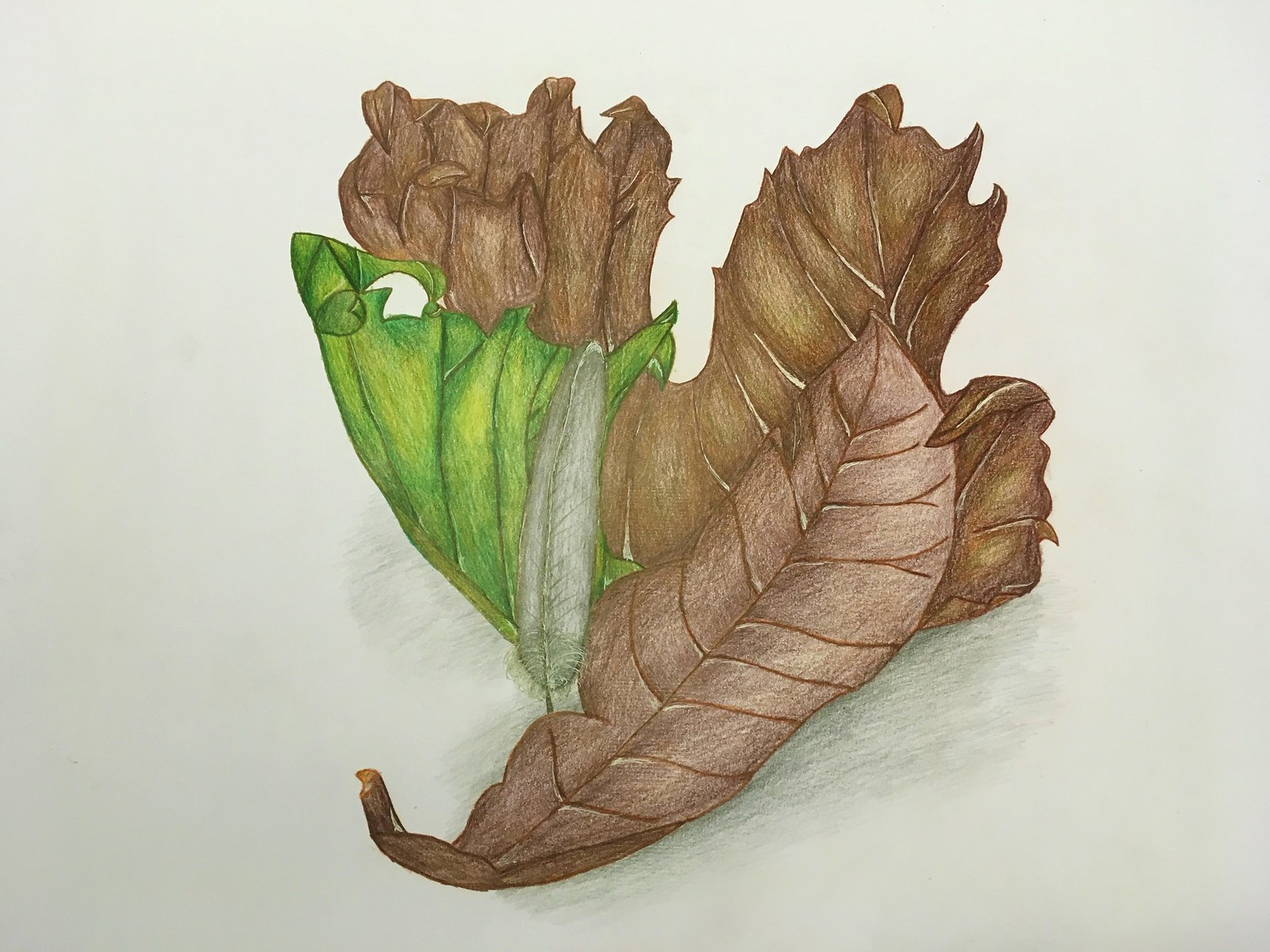This finely detailed image, likely created with colored pencils on a very light gray paper, features three meticulously rendered leaves at its center, showcasing a superb use of shading and shadows to impart a sense of dimension. The central focus is on the largest leaf, which has an oblong shape and a rich brown hue, indicative of an autumn leaf that has dried. The intricate brown veins add to the lifelike quality of the depiction.

To the right of this leaf is another, still green and possibly representing a silver maple based on its shape, although viewed from the side. This leaf is artfully rendered with varying shades of green and contrasting touches of yellow, enhancing its vividness. Behind this green leaf, a beautifully rendered maple leaf is visible. This third leaf has also dried, characterized by its range of brown shades, adding depth and realism to the overall composition.